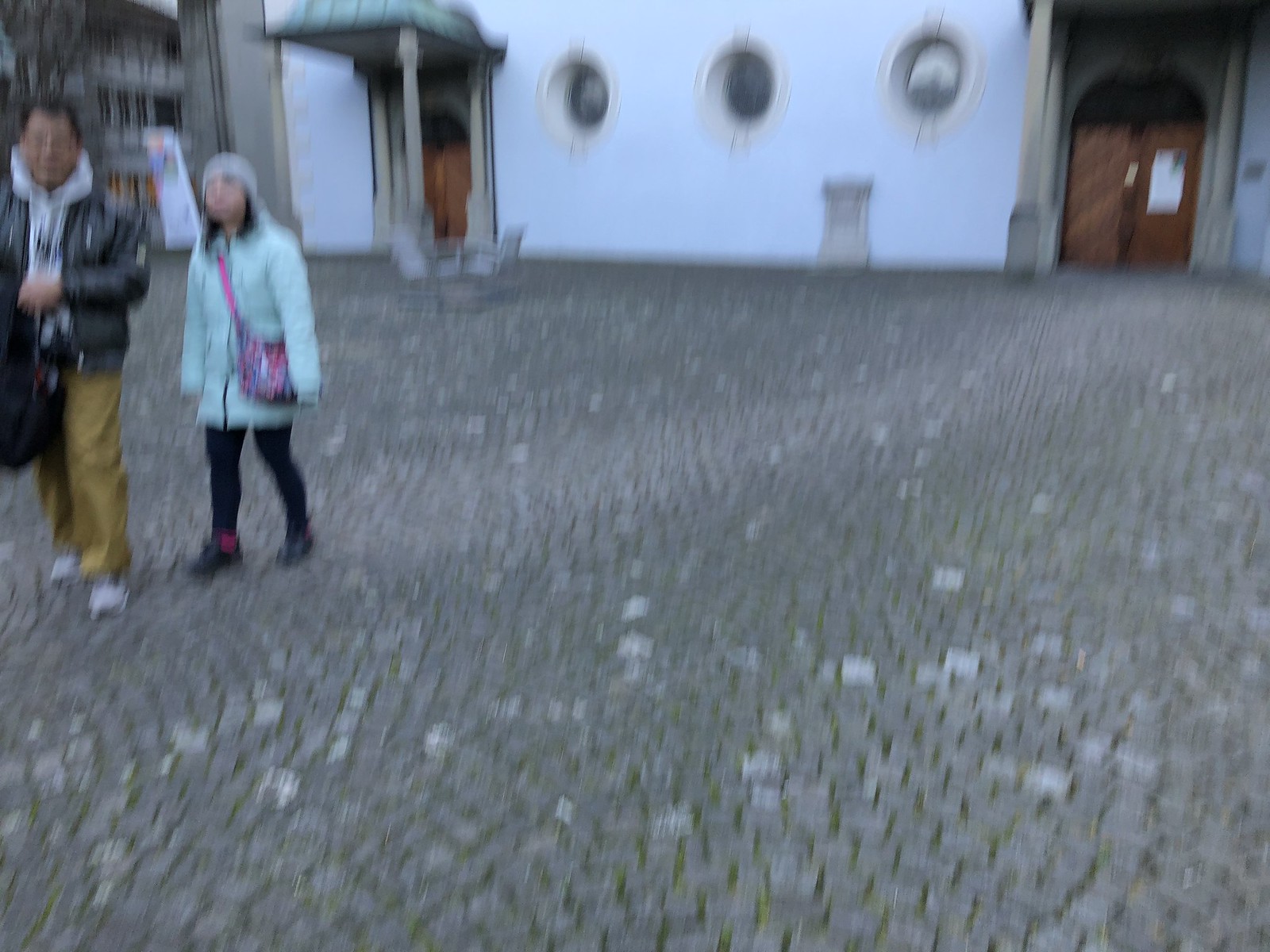This image portrays a somewhat blurry, distorted view of a paved plaza in front of a white building that features distinctive round windows and two wooden doors on either side. The outdoor scene focuses primarily on a brick-style roadway where two people, an Asian man, and woman, are walking on the left side. The man, standing closer to the viewer's right, has black hair, light brown skin, and wears glasses. His outfit consists of a black leather jacket over a gray hooded sweatshirt, mustard yellow pants, and gray tennis shoes. He carries a black backpack in his right hand while his left arm is raised, also holding the backpack. To his left is a woman shorter than him, with black hair and light brown skin, wearing a light gray hat and a minty blue, almost light teal, long winter coat that puffs slightly and extends nearly to her knees. She pairs this with black leggings, black shoes, and burgundy socks. Her pink and purple purse is strapped across her body, resting on her left hip. Both figures are positioned against the backdrop of the gray-bricked plaza, enhancing the serene and casual essence of the outdoor setting.